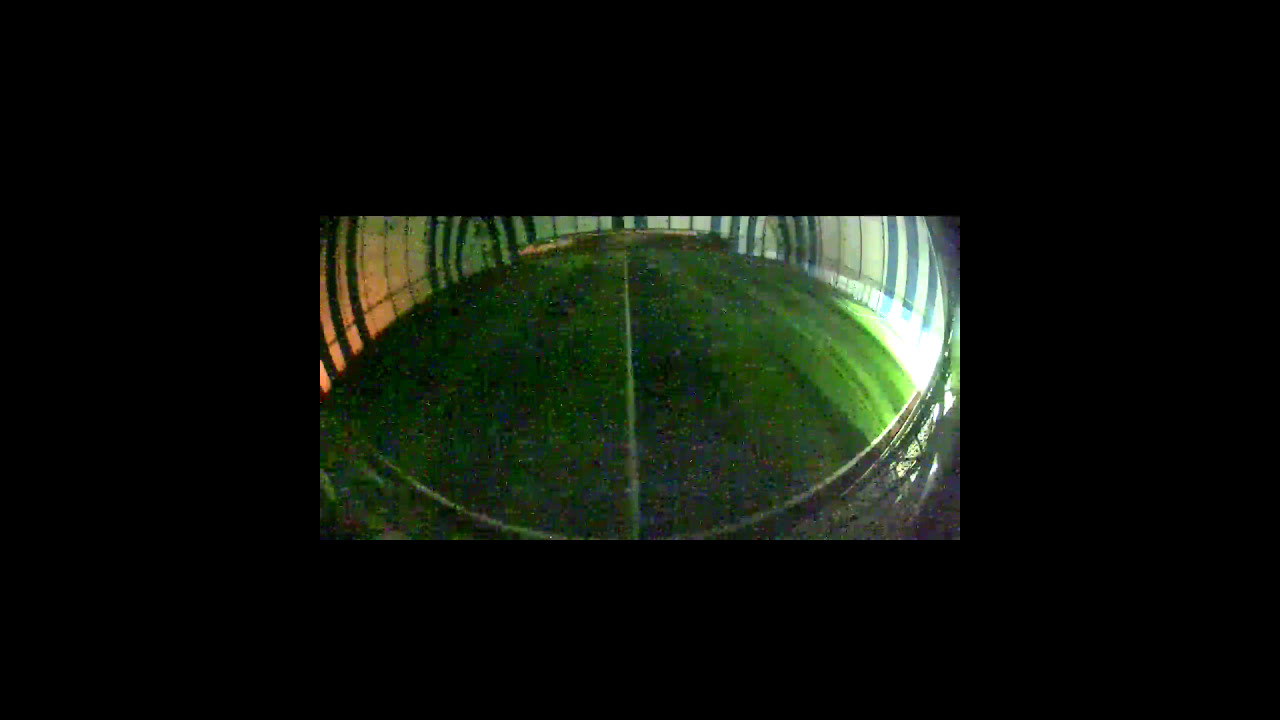The photograph depicts an indoor, dome-shaped stadium with a circular layout. The central feature is a vibrant green grass field, meticulously bisected by a straight white line extending from the foreground to the background. Surrounding the field, the structure's walls are adorned with repeating blue and white vertical stripes, creating a distinct visual pattern. The blue stripes alternate in segments, each about three rows wide, interspersed with white stripes. The image captures a moment where bright light streams in from the far right side of the building, enhancing the vividness of the grass in that area. A metal framework with intersecting pieces can be seen in the foreground, possibly part of a seating or structural arrangement. The entire scene has a prominent black border larger than the image itself, emphasizing the focal point within.